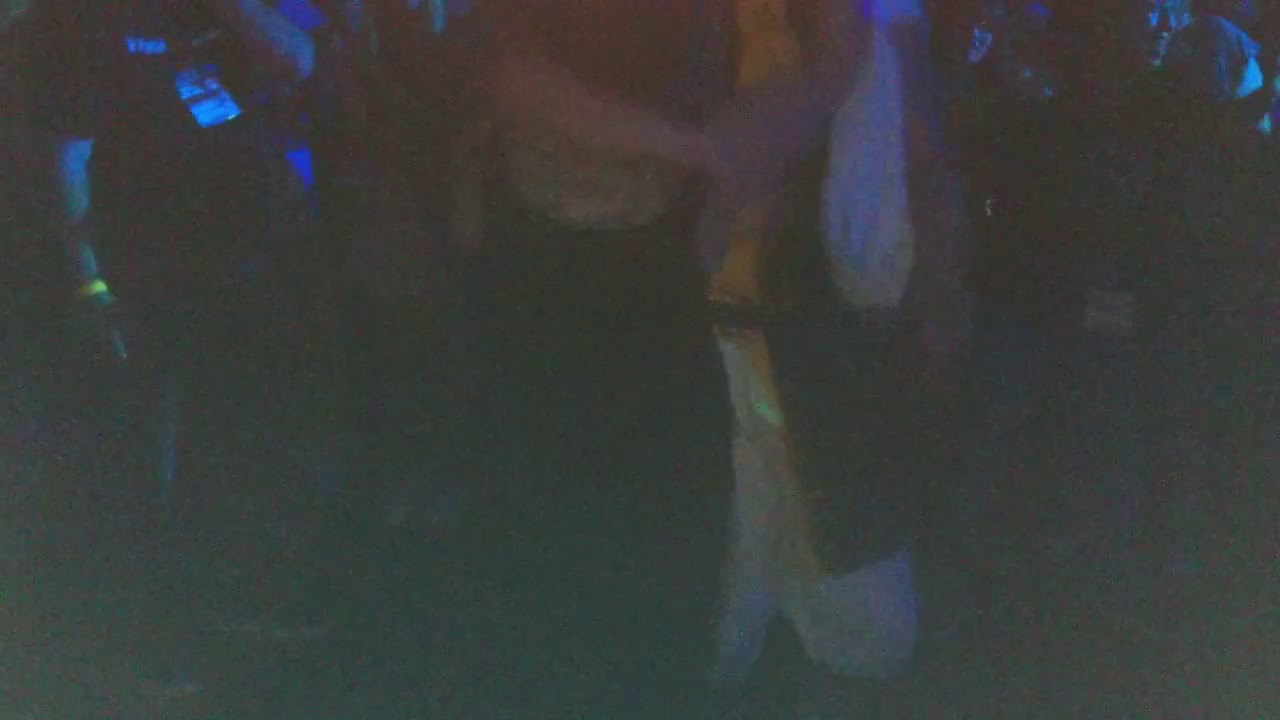The image is a very blurry, low-resolution photo taken in a dark setting possibly at a party, concert, or festival. The central figure is a gold, vertical, thin band of light with surrounding golden touches, making the scene even more difficult to discern. There seem to be two people in the middle, potentially hugging; one appears to be a woman in a black dress. A possible arm can be seen horizontally across the top left, with other figures to either side, dimly lit by blue light. Faces are barely discernible, with two faint, bluish faces visible in the background on the upper right. The left side features a gold band about a centimeter thick. Overall, the image is a blend of fuzzy gray and blurred forms, making identification challenging.